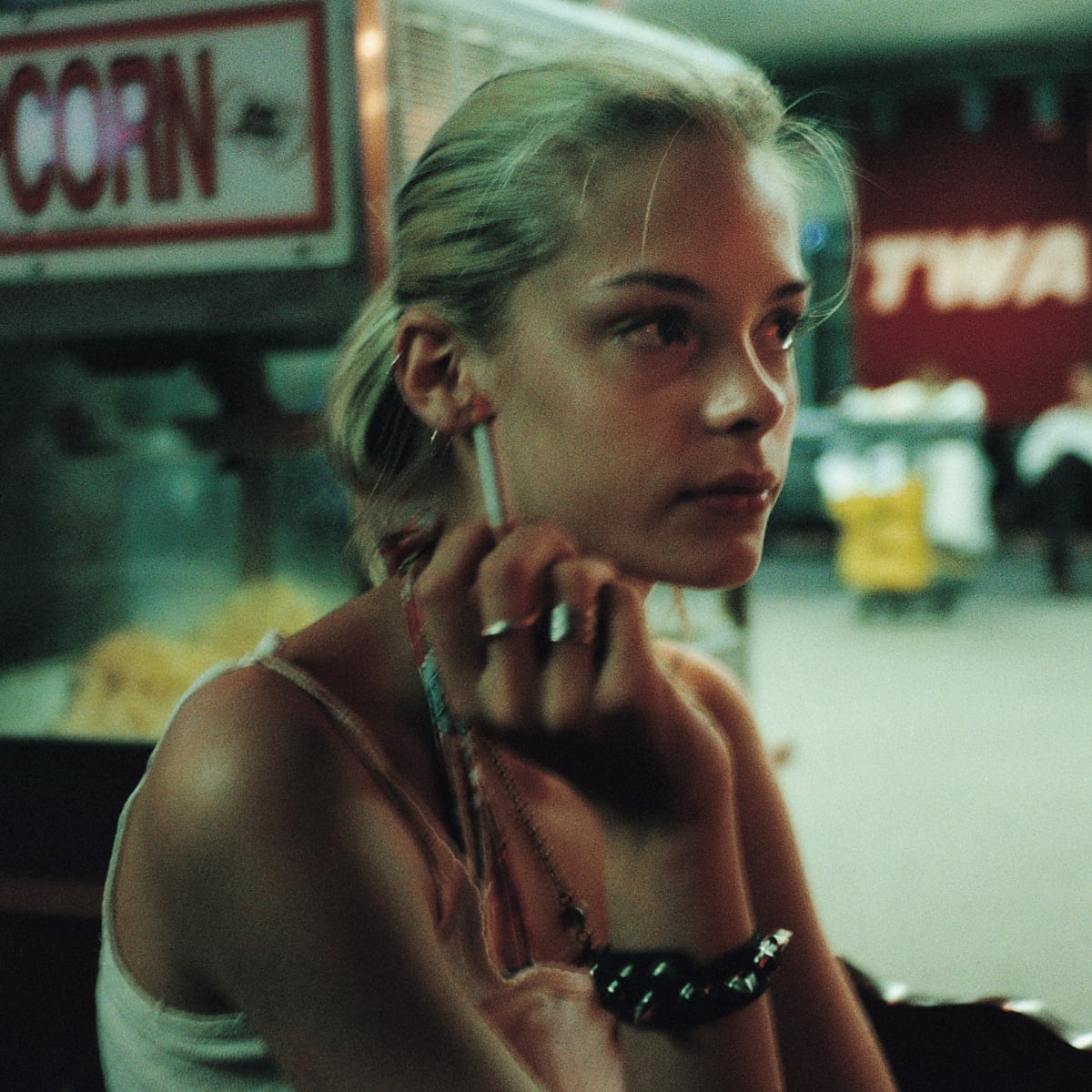In this grainy, cinematic photograph, a young Caucasian woman with long blonde hair pulled back in a ponytail sits, exuding a dramatic and nostalgic vibe. She holds a cigarette delicately in her right hand, with an assortment of rings adorning her fingers. Her serious expression is accentuated by her thick, dark eyebrows as she gazes off to the side. Dressed in a white spaghetti-strap tank top, she accessorizes with a black leather bracelet studded with silver spikes and multiple earrings in her right ear. The background features a red wall with the partially visible text "TWA" and a slightly out-of-focus popcorn machine, enhancing the vintage feel of the image with its filmic grain and soft, cool-toned lighting. The combination of these elements creates a scene that looks like a still from a bygone-era movie, impeccably captured to evoke a sense of timelessness and depth.